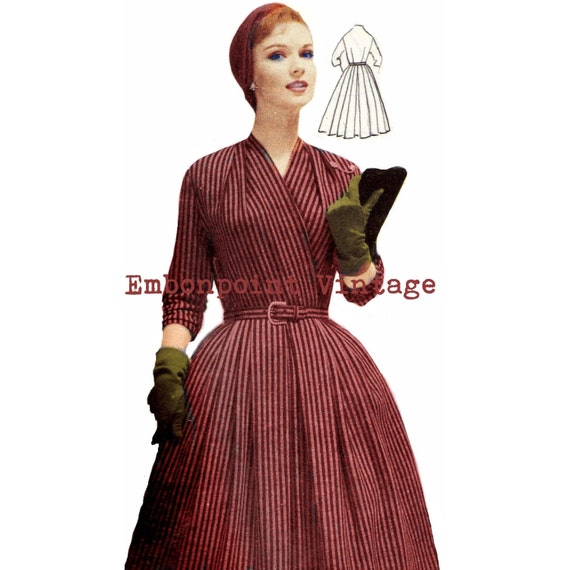This image is a vintage advertisement for a women's dress, possibly a sewing pattern, under the brand name Embonpoint Vintage. The central figure is an elegantly dressed woman, whose bright blue eyes contrast vividly with her meticulously styled red hair and subtly applied makeup. She is wearing a burgundy red dress adorned with lighter vertical stripes and featuring a tight waist belt. The dress has three-quarter sleeves, and she pairs it with olive green suede gloves that extend just above her wrists. Her accessories include a matching red cloth hat and a black clutch purse held to her chest. The background is predominantly white, emphasizing the woman and adding a sophisticated, clean aesthetic. Behind her, a drawing of the back view of the same dress hints at its design details, further suggesting this could be a pattern cover. The label "Embonpoint Vintage" is prominently displayed, matching the dress's burgundy hue, adding to the cohesive and stylish presentation.